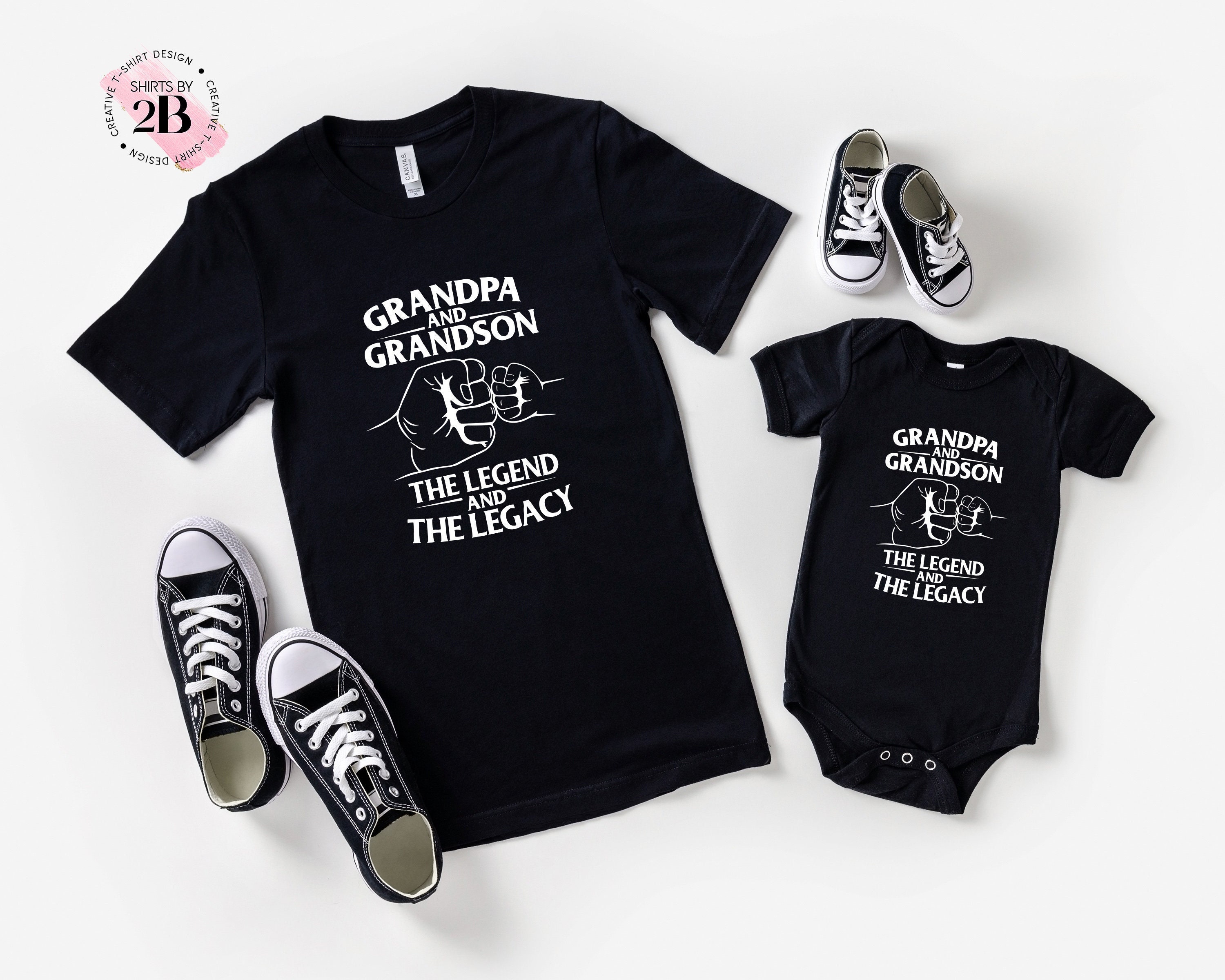This image is a professional advertisement, likely intended for an online shopping website, showcasing matching family clothing. Set against a white background, the photograph features a black adult t-shirt and a black infant onesie. Both garments have white printed text that reads "Grandpa and Grandson" above a graphic of a large fist bumping a small fist, and then "The Legend and the Legacy" below the graphic. Accompanying the clothing are two pairs of black and white casual shoes: a larger pair for the adult t-shirt and a smaller, baby-sized pair for the onesie. The top left corner of the image displays the logo of the selling company, "Shirts by 2B," encircled by the phrase "Creative T-Shirt Design" and marked with a thick pink stripe resembling a paint smear running diagonally across the logo.